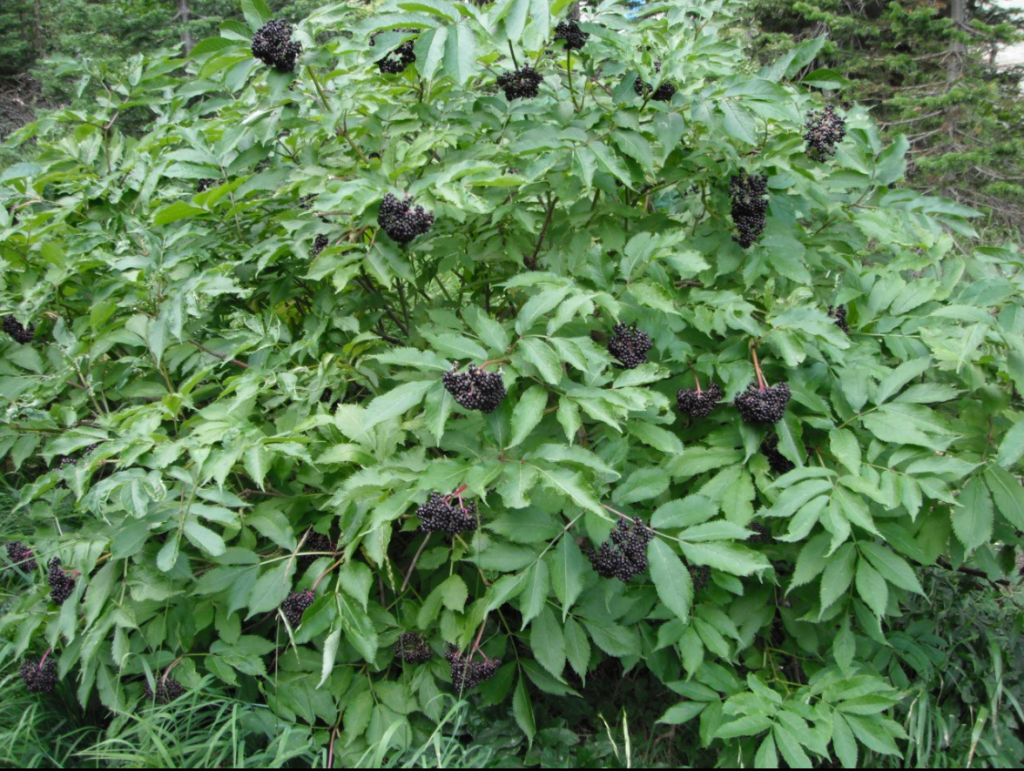The image captures a vibrant bush teeming with life, likely photographed during the day. Dominated by lush, green leaves, and healthy-looking stems, the scene is bursting with greenery. At the center of attention are several clusters of dark, purplish-black berries, which resemble blackberries. These berries, grouped in bunches of 5 to 6, dot the bush generously. The bush itself is low to the ground, surrounded by grass, and possibly some moss. While it is unclear whether the berries are edible or if the shot was taken professionally, the photo provides a crisp, detailed view of the shrubbery and its backdrop, which includes towering trees and a snippet of natural forest floor. No animals or people are visible, making the bush and its berries the main focus of this serene, nature-filled setting.